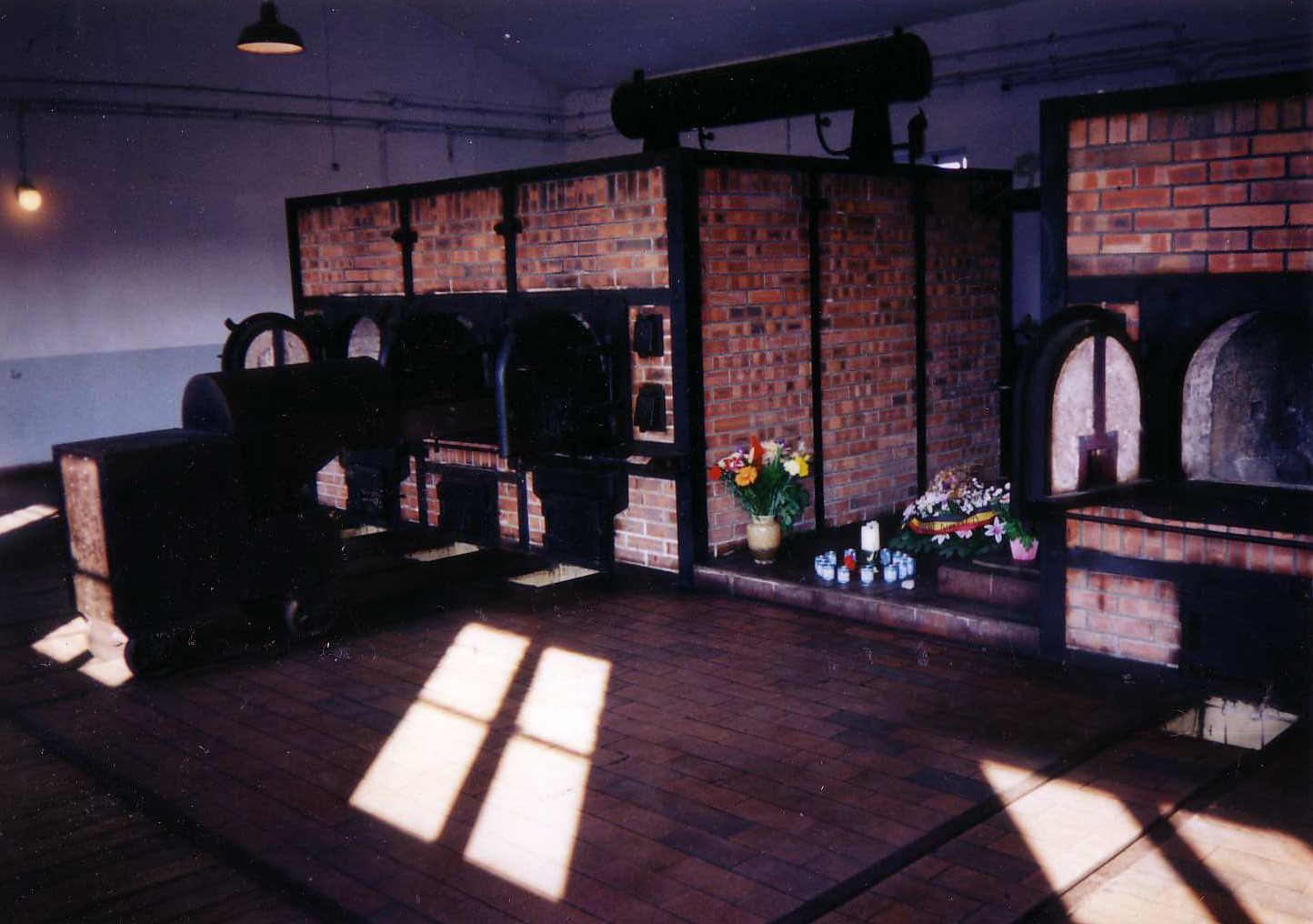The photograph depicts a dimly lit interior of a brick building, possibly a morgue or crematorium, characterized by its shadowy and minimal lighting. Dominating the scene are two brick structures with a three-dimensional rectangular shape, reminiscent of ovens or pizza ovens, situated on a wooden floor. Both structures feature cylindrical openings—one fully visible on the left and the other partially visible on the right—each with three doors. The orange bricks are accented with black wooden design elements. The setting is illuminated by patches of sunlight filtering through the silhouette of rectangular windows, casting a parallelogram-shaped shadow on the floor, suggesting it is daytime. Control panels are seen on the right side of the left structure, with a noticeable fluorescent light fixture overhead. In the hallway between the structures, flowers are visible, possibly lying on the ground. The backdrop consists of a white and gray wall, further emphasizing the stark and solemn atmosphere of the room.